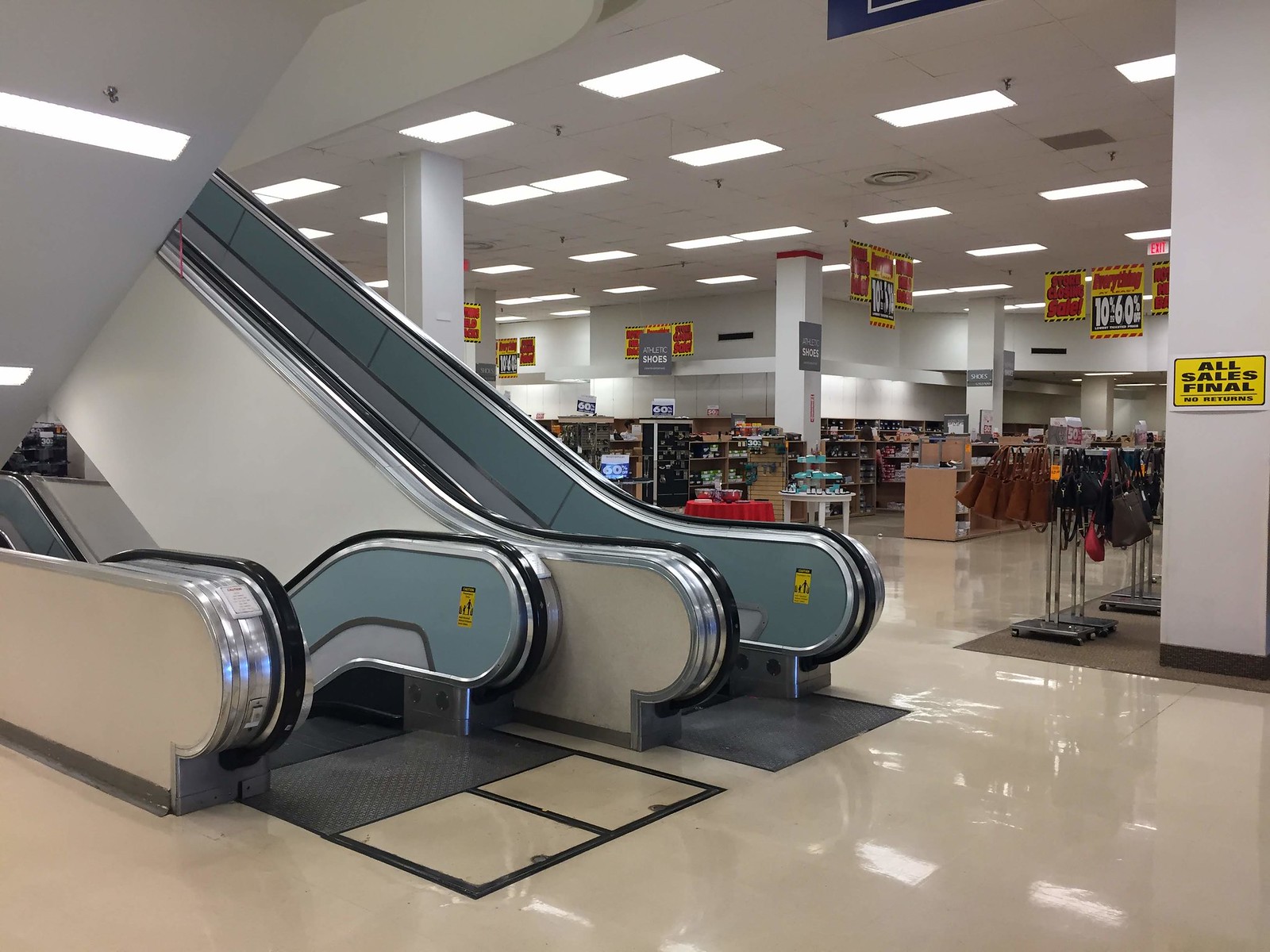This image captures the interior of a department store, focusing centrally on two escalators—one ascending and one descending. The store appears to be undergoing a significant closeout sale, evidenced by numerous "All Sales Final" signs and discounts ranging from ten to sixty percent. The photograph, taken in a landscape format from the perspective of a person standing on the floor, highlights the store’s meticulous cleanliness, with its shiny, wax-coated off-white floors and bright fluorescent lighting reflecting off the surfaces.

The escalators, positioned to the left in the image, have gray paneling, slate blue and gray interiors, and glossy black railings. Yellow caution signs are attached to them, and black mats are present at both the entry and exit points, surrounded by black floor squares. The store's layout features various items, notably handbags and possibly shoes, displayed on racks and round tables. The ceiling is supported by white pillars and adorned with rectangular light fixtures, enhancing the spacious and well-lit environment. The overall atmosphere suggests a large, somewhat upscale department store, reminiscent of a Zeller’s or The Bay.